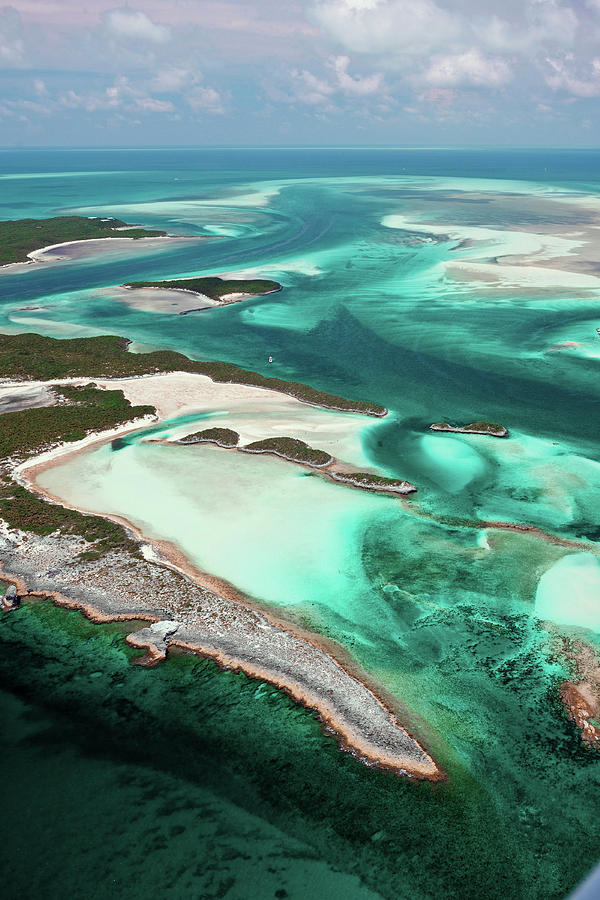This aerial photograph captures a stunningly vibrant, aqua blue and turquoise ocean, most likely characteristic of a tropical region such as the Caribbean. The portrait-oriented image offers a breathtaking view of multiple small islands and inlets scattered throughout the serene waters. A significant land formation occupies the left side, stretching towards the bottom right with a narrow, sliver-like shape. Its surface is predominantly gray gravel, transitioning into a light pink rocky beach with a border of dark green trees. The upper portion of this island's border curves around to the right, forming a picturesque bay with a pristine white sandy beach and a shallow ocean area, revealing the white sandy floor beneath. The water, rich in color, seems to hold patches of coral or seaweed, adding to the natural beauty of the scene. The horizon is set about a quarter of the way down the image, displaying an expansive sky filled with puffy white clouds. The overall sense is one of untouched paradise, devoid of any human presence, infrastructure, or identifying markers, leaving the viewer to marvel at the pure, unspoiled elegance of the landscape.